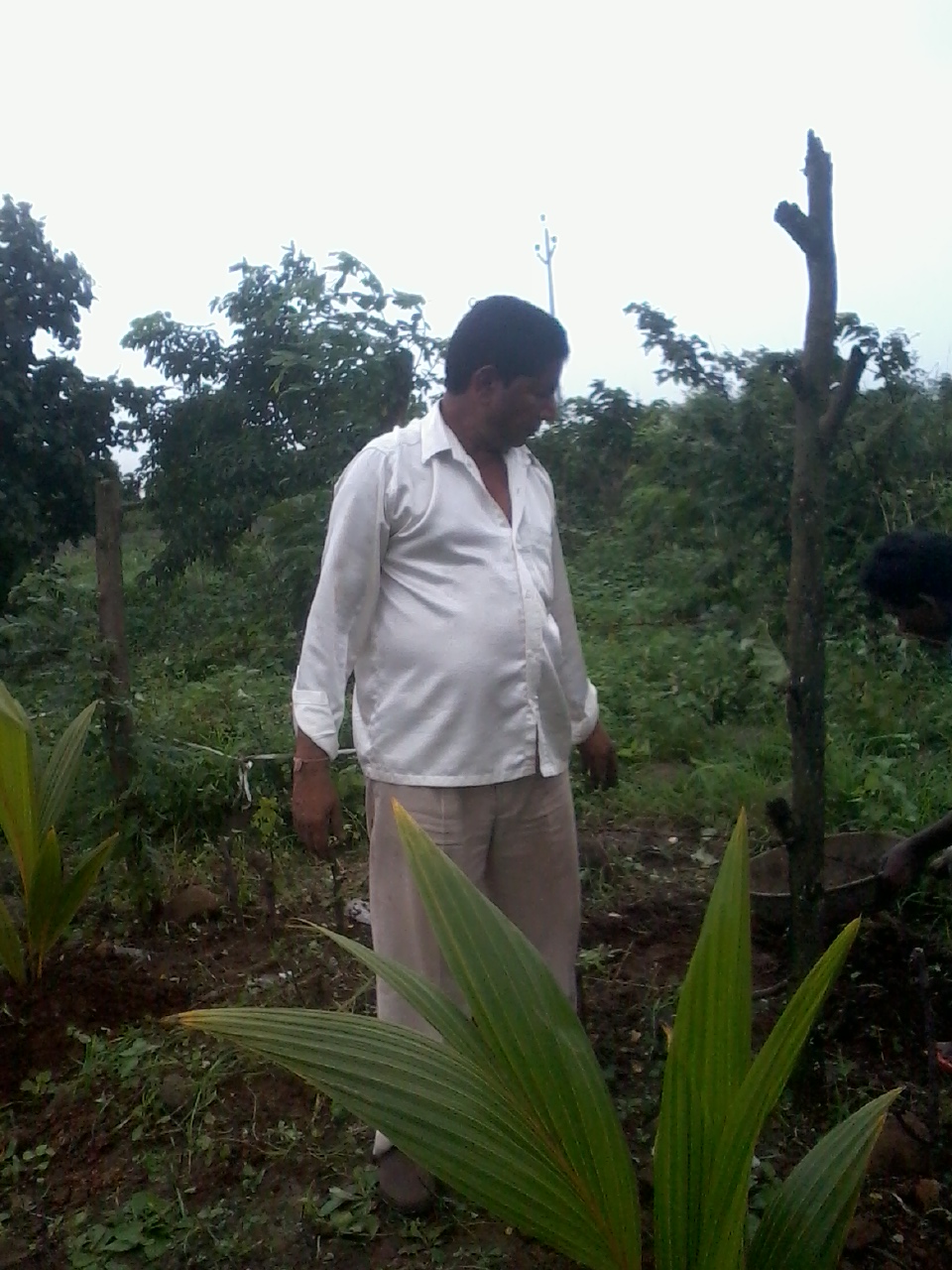A middle-aged man with dark skin and dark hair stands in a lush garden or possibly his backyard, surrounded by a mix of wild and cultivated plants. He is wearing a white silky, long-sleeved button-down dress shirt, slightly unbuttoned at the top and bracelet on his wrist, khaki-colored baggy pants, and brown shoes. The sky above is white, and it is daytime but not particularly sunny. The man is looking down and to his right, examining the soil and large green plants with enormous leaves, possibly ferns or aloe, some of which resemble palm leaves. In the background, a large, bare tree trunk without branches or leaves stands prominently among green grass, shrubs, and taller trees. Also present, though partially visible, is another individual, likely a woman holding a wooden basin, hinting at a shared activity or task within this verdant setting. Scattered gray rocks add texture to the earthy surroundings, emphasizing the natural and unmanicured look of the garden. The overall scene gives an impression of a casual, unprofessional snapshot capturing a moment of quiet admiration and labor in a lush, green environment.